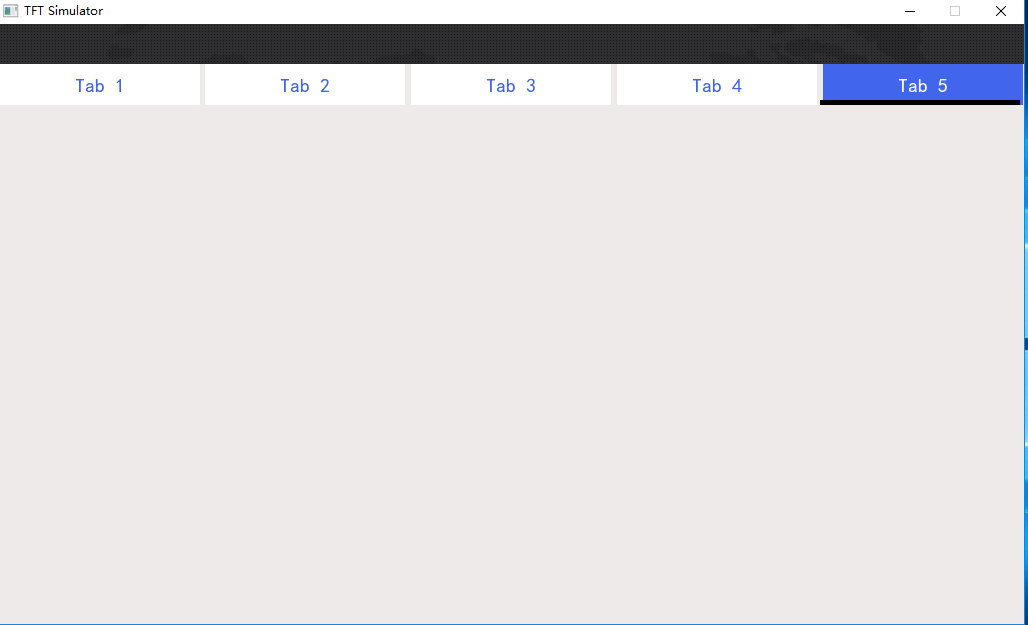This cropped screenshot features a panel from an application titled "TFT Simulator," as indicated by the small black text in the top-left corner. Directly below this title is a prominent black rectangular bar extending across the entire width of the image. Underneath the bar are five horizontal tabs, each styled as white rectangles with blue text. The tabs span from the left to the right side of the screen, with the fifth tab distinctly highlighted in blue. The gray area beneath these tabs is unmarked and void of any text or additional elements. Noticeable imperfections in the cropping are present; the left side of the image is unevenly trimmed, cutting off a portion of the leftmost tab and displaying jagged blue edges. Additionally, a faint blue line can be observed at the bottom of the image, whereas the top of the screenshot appears to be cropped, as any line above the app's interface is out of view.